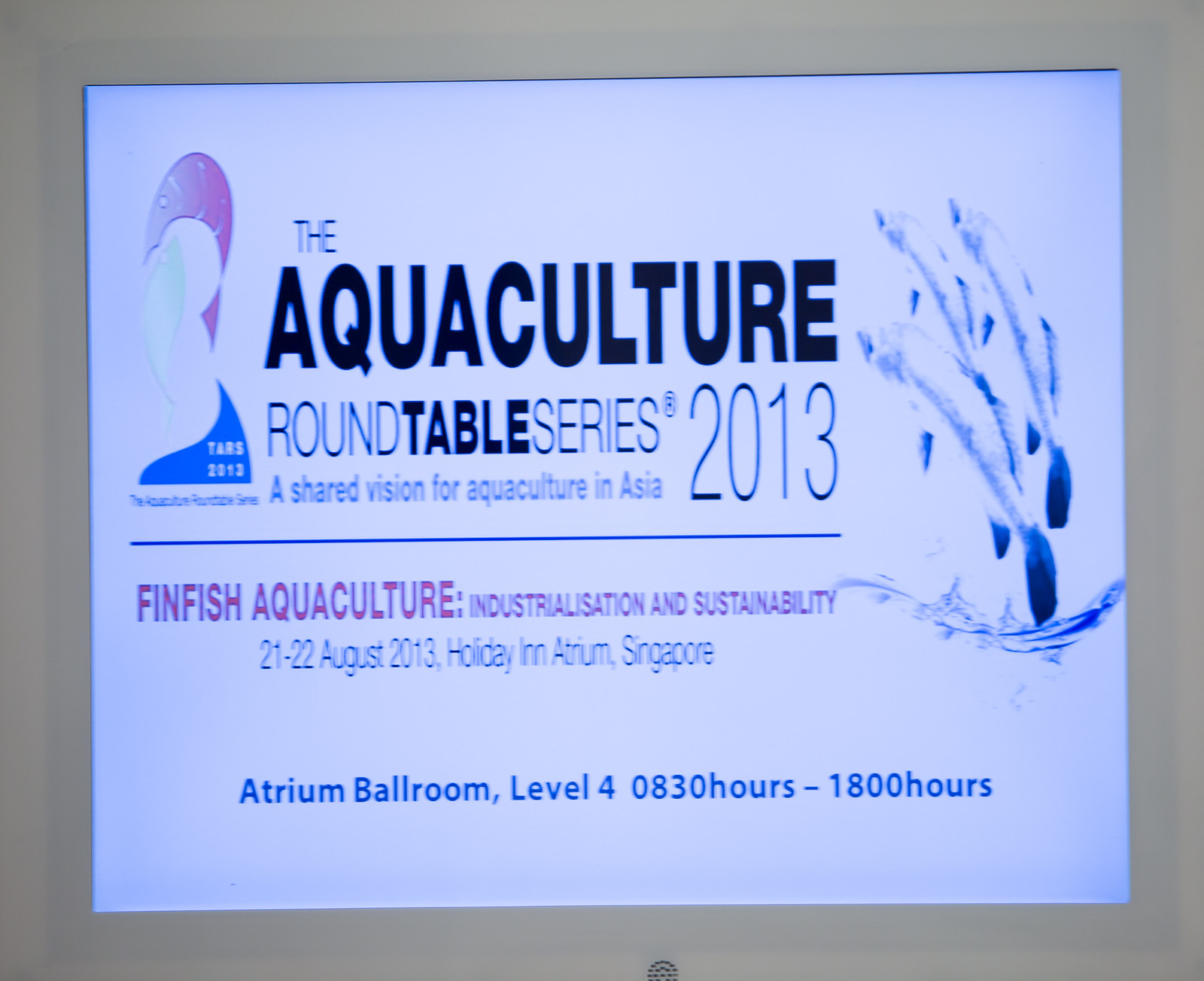In the center of this indoor image, a white projection screen or monitor displays a detailed presentation slide with an off-white background. The slide prominently announces the "Aquaculture Roundtable Series 2013: A Shared Vision for Aquaculture in Asia." The text is in black, with three trout jumping out of the water on the right and a small fish logo in the upper left corner labeled "TARS 2013." Further details on the slide read "FinFish Aquaculture Industrialization and Sustainability," while the event specifics note "21 to 22 August 2013, Holiday Inn Atrium, Singapore," and list "Atrium Ballroom, Level 4, 0830 hours - 1800 hours." The slide's appearance suggests it is being projected for a presentation, and possible blurriness indicates the image might have been taken while the photographer was in motion.